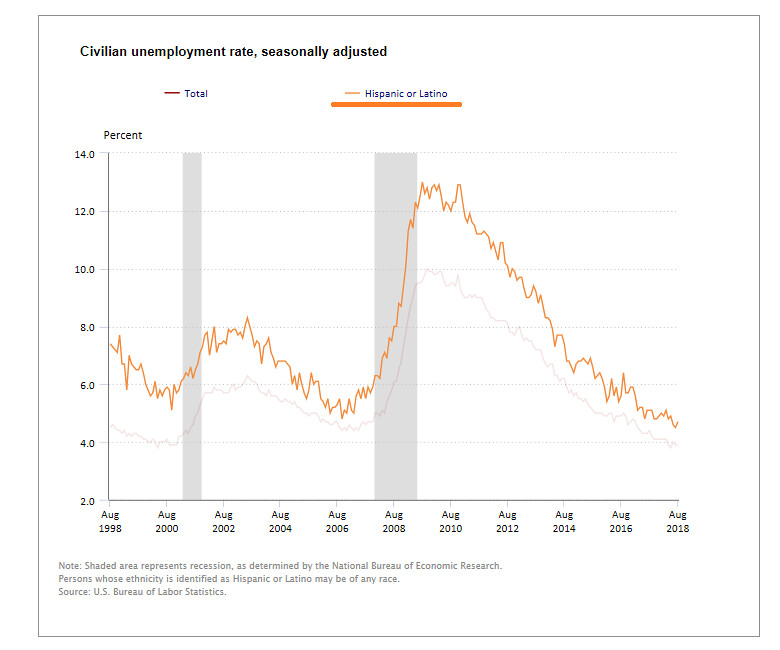The image features a graph titled "Civilian Unemployment Rate, Seasonally Adjusted" with a simple white background and a thin black-gray frame. The graph spans from August 1998 to August 2018, with the horizontal axis representing time and the vertical axis ranging from 2.0% to 14.0% unemployment. The data is split into two lines: a red line for "Total" unemployment and an orange line depicting the "Hispanic or Latino" unemployment rate. Both lines exhibit considerable fluctuations, with the orange line starting just below 8%, dipping below 6%, rising past 8%, and peaking around 13% in August 2010 before gradually descending to just above 4% by August 2018. Notable details include a highlighted note at the bottom of the graph indicating that shaded areas represent recessions, as determined by the National Bureau of Economic Research, and clarifying that individuals identified as Hispanic or Latino may be of any race. The source for the data is cited as the US Bureau of Labor Statistics.